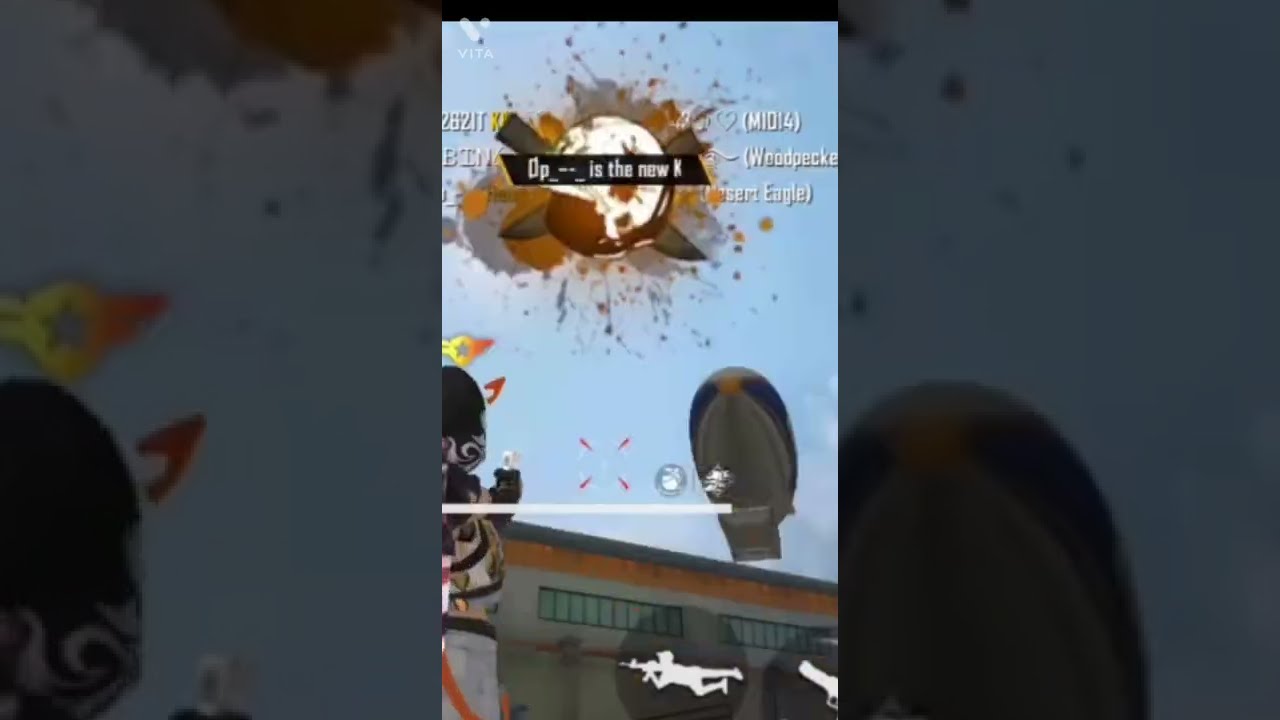The image is a blurry, low-quality screenshot from a third-person shooter video game, captured with a phone in portrait style. The game scene is stretched horizontally, bordered by dark gray filters on the sides. At the center of the frame, a player character dressed in black and white is located in the bottom left corner, holding a pistol. Above them, an explosion is depicted with a white core and brown and gray splashes, resembling two crossed knives or a skull and crossbones with an exploding ball on top.

In the sky, a gray blimp with blue sides flies towards the explosion near a building characterized by cement walls, thin warehouse-style windows, and a flat roof. Along the bottom of the image, there is a silhouette of a man crawling with a sniper rifle. The game's HUD elements and icons are visible: white text on the screen includes "zbizit btn desert eagle woodpecker midi4" and "0p is the new K."